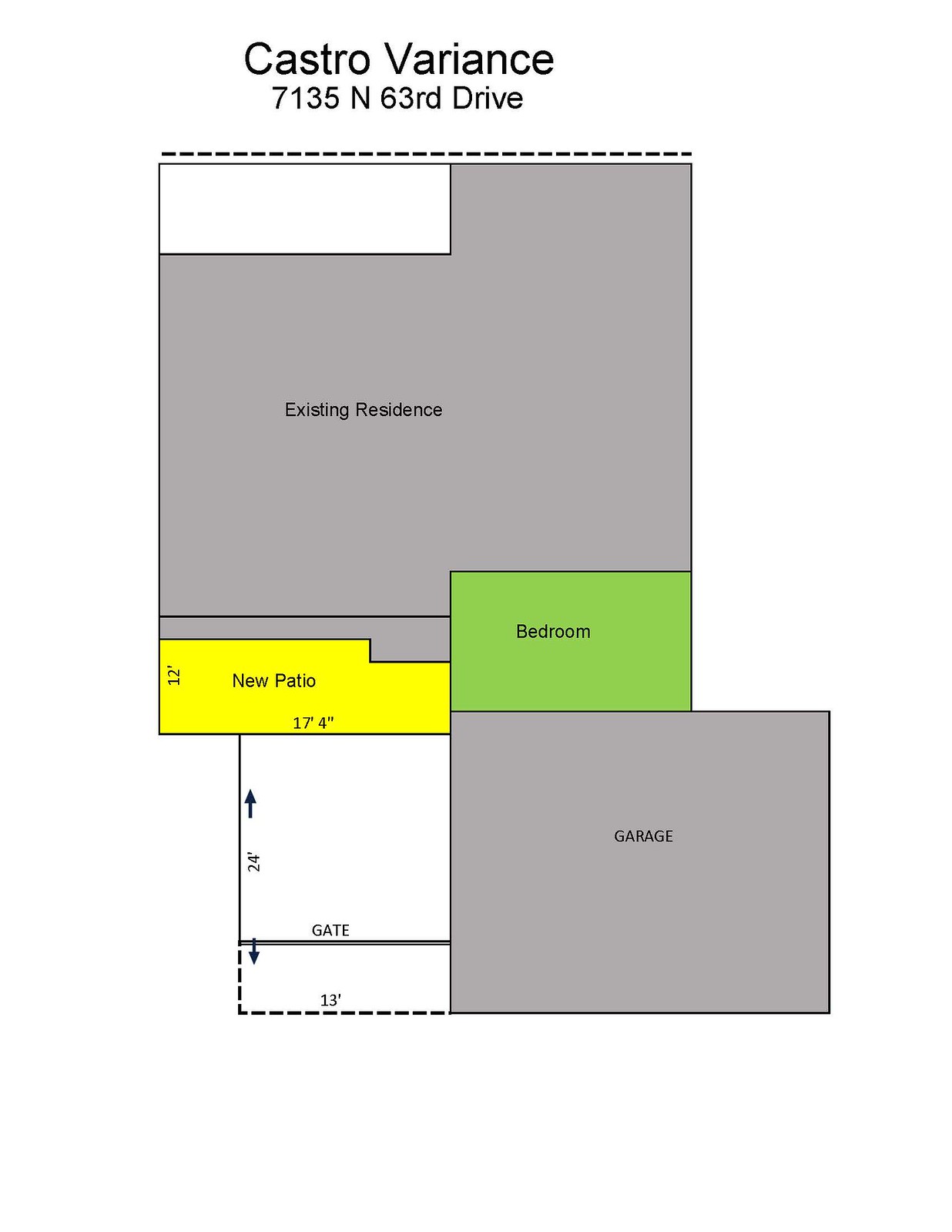This detailed blueprint outlines the layout of a residential property located at 7135 North 63 Drive, labeled at the top as "Castro Barayens." The blueprint displays various sections of the property, identified with precise terminology. At the top center, it specifies the "Existing Residence," represented by a large square area. Below this main residence area, there is a designated "Bedroom" to the right and a newly added "Patio" adjacent to it. Directly beneath these sections, the blueprint shows the "Garage," which is situated centrally. To the left of the garage, the entry "Gate" is marked. The blueprint is meticulously divided, with clear lines demarcating each space within the overall layout, providing a comprehensive overview of the property's design and structure.